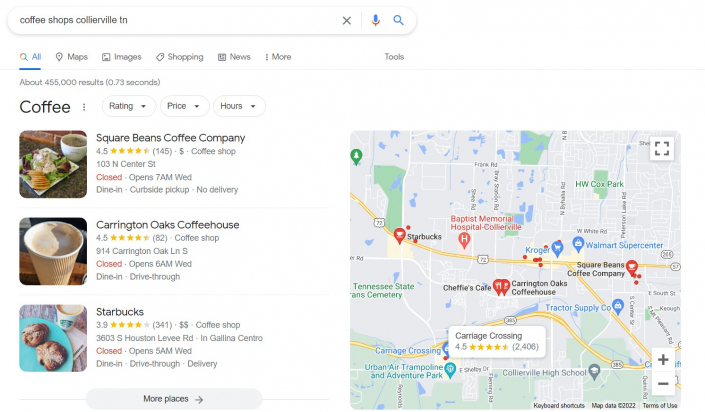**Screenshot of Google Search Results for Coffee Shops in Collierville, Tennessee**

This image captures a Google search results page with a clean white background. At the top left is a rounded search bar with a subtle light gray shadow. Inside the search bar, the query "Coffee shops in Collierville, Tennessee" is typed in black text. Adjacent to the search bar on the right, there's some negative space followed by a gray 'X', a thin vertical light gray line, a multicolored microphone icon, and a blue magnifying glass icon.

Below the search bar are various tabs starting with a multicolored magnifying glass icon followed by the word "All" in blue, highlighted by a blue underline. The subsequent tabs are in gray: 
- A geolocation pin icon with the text "Maps."
- A picture icon with the text "Images."
- A shopping tag icon with the text "Shopping."
- A newspaper icon with the text "News."
- Three vertically stacked gray dots labeled "More."

To the far right, there is the gray word "Tools" with no accompanying icon. 

A thin gray line with a blue underline separates the tabs from the main body of the page below, which also has a white background. 

At the top of the results section, light gray text states "About 455,000 results (0.73 seconds)" on the left, justified. Below it, large black text reads "coffee," followed by three vertically aligned gray dots and three pill-shaped buttons. Each button has thin light gray outlines and is filled with white. Inside the buttons are the words "Rating," "Price," and "Hours," each followed by a black downward arrow.

Beneath this is a series of three listings, each separated by thin light gray lines. Each listing features a black title at the top and a square picture with rounded corners on the left side. There is also a large map on the right side of the listings.